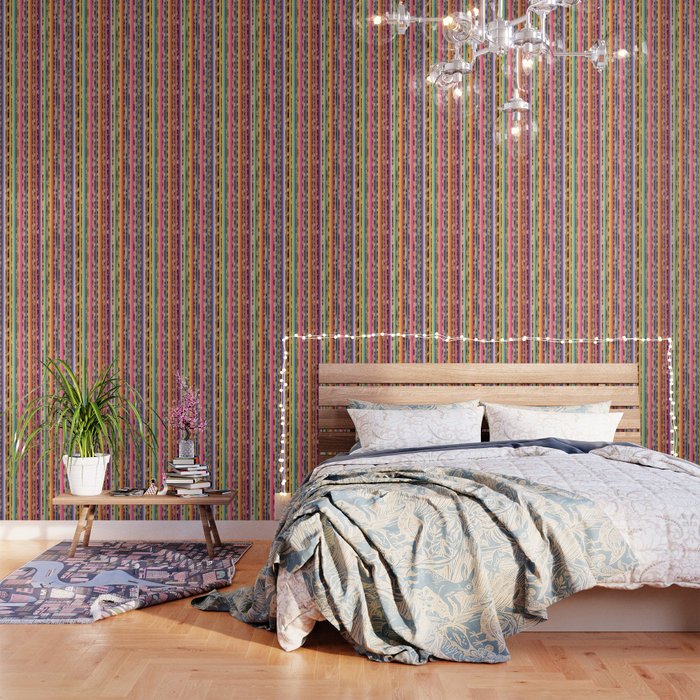The photo presents a large, somewhat sparsely decorated bedroom with a strikingly unique ambiance. The backdrop is dominated by a multi-colored, vertically striped wallpaper featuring hues like green, pink, and checkered patterns in black and orange, reminiscent of a rainbow-like appearance. This vibrant wall adds a lively contrast to the room. A contemporary, space-age silver chandelier with at least seven clear, circular enclosures containing visible bulbs hangs from the ceiling, adding a modern touch.

The bed, likely king-sized, sits prominently in the center, adorned with green sheets over cream-colored, fancy bedding with a subtle blue print, including an image of a rabbit jumping. It is surrounded by a series of horizontal slats forming the headboard, crafted from dark wood, and bordered by a string of rectangular Christmas lights, highlighting the bed frame.

On the left side of the bed, a small coffee table is positioned against the wall. This table displays a green, springy plant in a white container and a small silver pot with a pink plant. A haphazard stack of books and another silver container with a pink plant add to the eclectic decor. Below the table lies a pink rug, intricately designed to resemble a bird's-eye view of a town, featuring a street or stream amidst a variety of rooftops. The rug's corner is notably folded, possibly indicative of recent foot traffic or movement.

The overall aesthetic of the room blends modern and whimsical elements, captured in the scattered yet thoughtful placement of its furnishings and decorations.